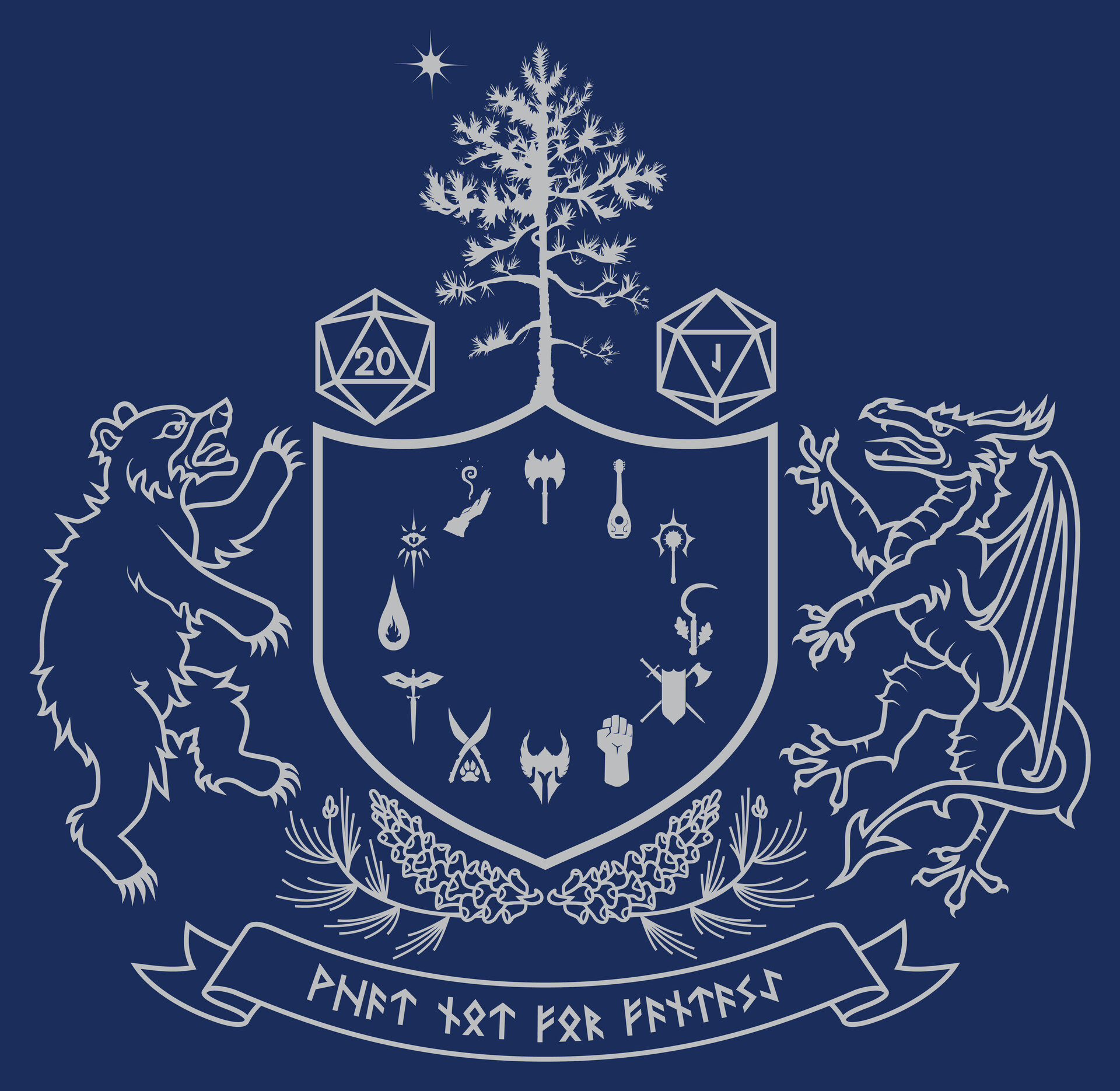This image showcases a meticulously detailed coat of arms set against a dark blue background, likely inspired by Dungeons and Dragons. At the top of this white-outlined crest, there stands a small white tree, flanked by two twenty-sided dice. One die shows a "20" while the other displays a "J." The crest is crowned by a dragon on the right and a fierce bear on the left. 

Inside the shield, various symbols representing elements of warfare and character classes from Dungeons and Dragons are densely packed. These include a double-sided battle axe, a mandolin, swords, fire, armor, and a shield, among others. Below the shield, a laurel or wheat motif is split and extends outward on both sides, signifying achievement or honor.

Under this laurel, a banner bears mysterious inscriptions—possibly "PNFT, XRX"—in a language that is not immediately recognizable. This detailed crest evokes imagery of both fantasy and heraldry, akin to an insignia for a fantastical realm or guild.